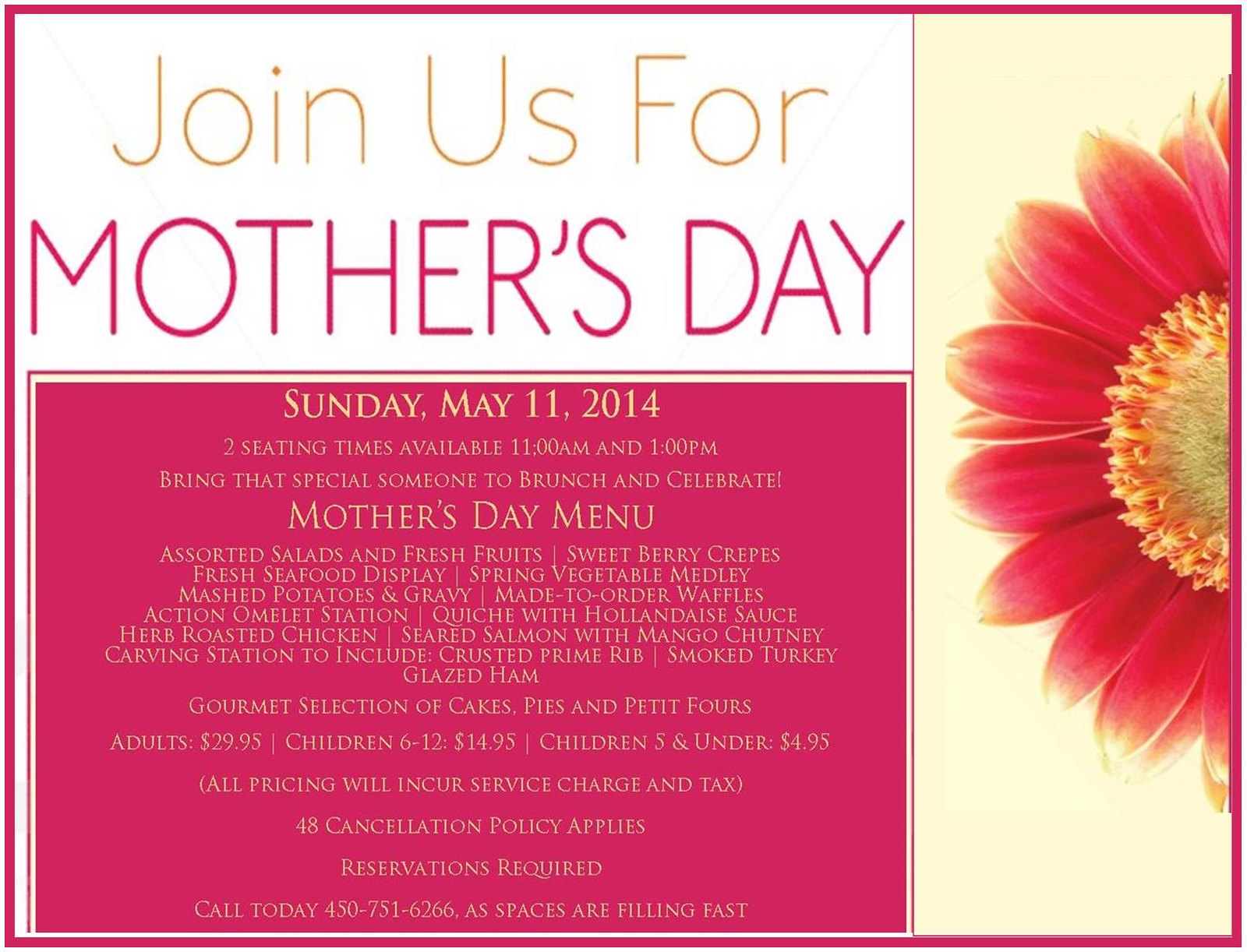This image is a rectangular promotional poster for a Mother's Day brunch event, slightly wider than it is tall, with a thin bright pink border encircling it. The poster is divided into three parts. 

On the right side, occupying about one-fourth of the width, there's a background of light tan or yellowish color featuring a striking half-image of a red flower with yellow-tipped petals and prominent yellow pollen areas. 

The left part of the poster is split horizontally into two sections. The top section has a white background with faint diagonal light blue stripes, and features thin gold text that reads, "Join us for," followed by bold pink text stating, "Mother's Day." 

The bottom section has a mix of light tan and pink backgrounds. Here, a bold message reads, "Sunday, May 11th, 2014. Two seating times available 11 a.m. and 1 p.m. Bring that special someone to brunch and celebrate." 

The detailed Mother's Day menu includes: assorted salads and fresh fruits, sweet berry crepes, fresh seafood display, spring vegetable medley, mashed potatoes and gravy, made-to-order waffles, action omelet station, quiche with hollandaise sauce, herb-roasted chicken, seared salmon with mango chutney, and a carving station with crusted prime rib, smoked turkey, and glazed ham. It also mentions a gourmet selection of cakes, pies, and petit fours. 

Pricing details are: adults $29.95, children ages 6 to 12, $14.95, and children 5 and under, $4.95. All prices incur a service charge and tax. Additionally, a 48-hour cancellation policy applies and reservations are required. The poster suggests calling 450-751-6266 soon as spaces are filling fast.